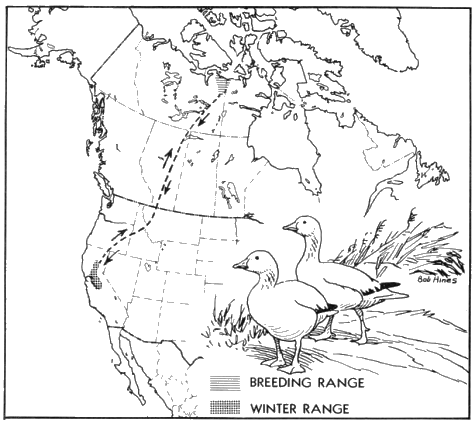This black and white illustration is a detailed map of the continental United States, displaying the migration path of geese. The map emphasizes two geese prominently occupying the right side, which are depicted facing westward toward the U.S. The line marked from California to Canada, accompanied by arrows pointing in both directions, delineates their migratory route. According to the map, the geese's winter range extends into mid to northern California, whereas their breeding range spans across Canada. Additionally, the bottom right corner features an artistic portrayal of the two geese amidst greenery, credited to artist Bob Hines. The map, devoid of color, has a scientific, analytical feel, underscoring regions unspecified by additional hues.